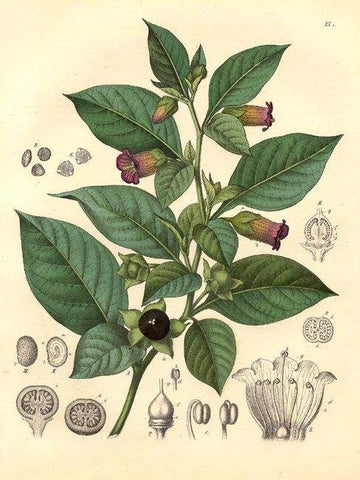This detailed vintage illustration depicts a botanical drawing of a plant, meticulously rendered in black and white ink and enhanced with subdued yet precise coloring. The plant features a robust green stem that branches out into approximately 12 or 13 tapered leaves of varying sizes, intricately showcasing delicate veins. Positioned against a white or slightly tanned background, this instructional image resembles those found in horticulture textbooks.

Near the plant's base, a black flower is fully bloomed, revealing its central seed, while near the top, three red flowers—two facing right and one left—are in full bloom, accompanied by a younger, not-yet-bloomed flower. This mix of foliage and flowers illustrates different stages of the plant's life cycle.

Surrounding the main illustration are smaller, uncolored diagrams—drawn in fine black ink—offering additional educational insights into the plant's cross-sections, stamen, pollinator parts, seeds, fruit, and early developmental stages. These supplementary illustrations provide a comprehensive understanding of the plant's anatomy and growth, contributing to the image's value as an educational reference.